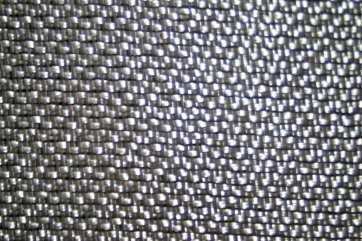This image presents an intricately detailed close-up of a piece of black mesh fabric, characterized by a remarkable interplay of textures and colors. The fabric is meticulously stitched in a horizontal pattern, creating a grid-like arrangement of small, well-defined black squares interspersed with silvery, whitish squares. The material exhibits a fine weave, reminiscent of chain mail or a similarly dense mesh, with sections appearing to weave in and out, lending a multi-directional flow to the pattern. A soft light illuminates the right side of the photograph, producing a subtle lens flare and highlighting the shiny, gray-black hue of the fabric. The overall appearance suggests a highly textured surface, almost as if composed of closely packed spheres that blend to form a nearly flat, tightly bound surface. The fabric, with its array of shadowed and lit sections, creates a compelling visual tapestry devoid of any background, focusing entirely on the complexity of the mesh itself.